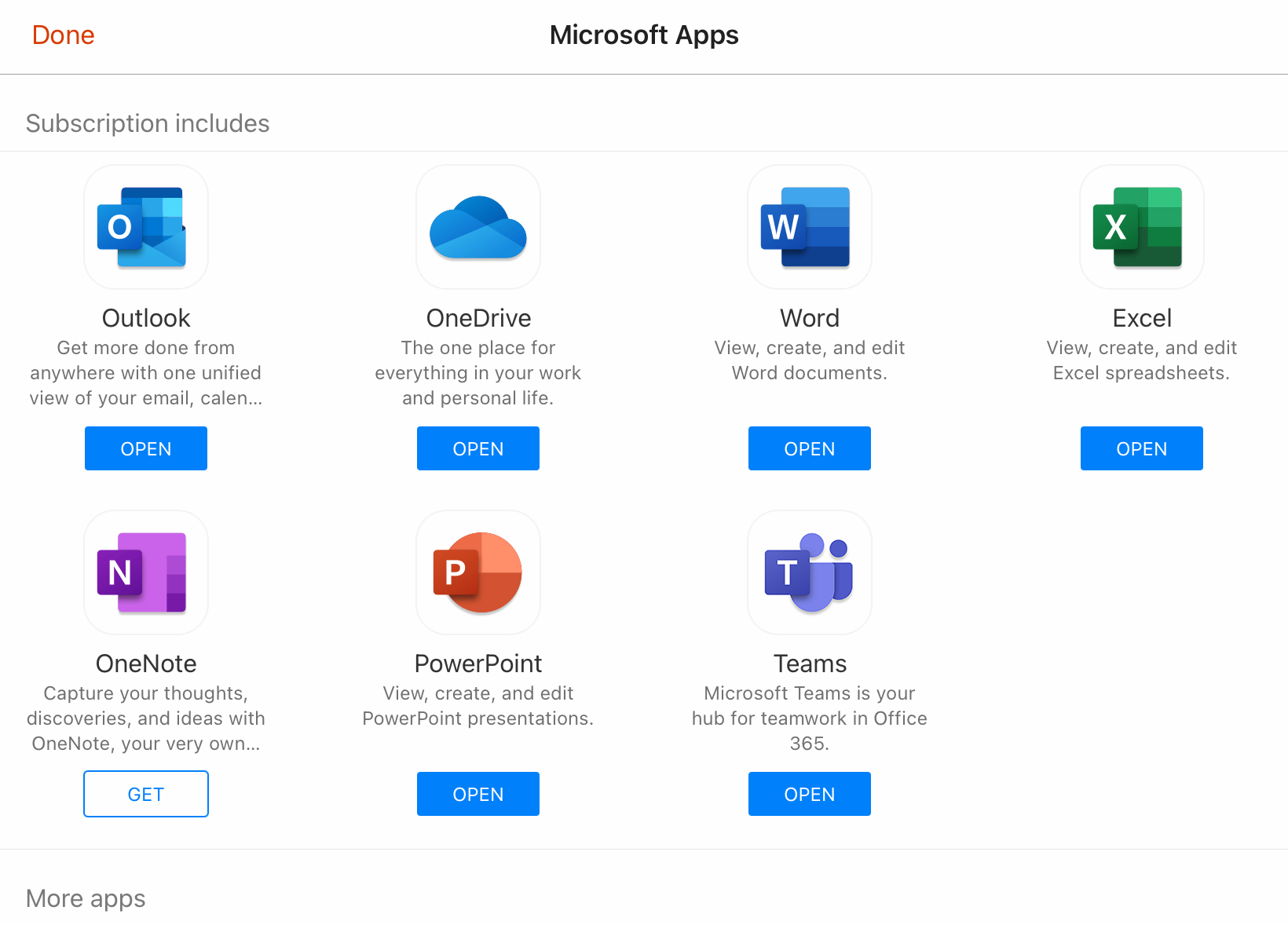This image is a screenshot of Microsoft apps, prominently featuring the title "Microsoft Apps" at the top center. On the left side in red, it says "Done," and just beneath that, in gray text, it reads "Subscription includes." Below this, the app list begins, starting with "Outlook," which states, "Get more done from anywhere with one unified view of your email and calendar..." Underneath Outlook, there is a button labeled "Open."

Next to Outlook, on the right, is "OneDrive," described as "The one place for everything in your work and personal life," with a blue "Open" button beneath it. Moving further to the right is the "Word" app, where it says "View, create, and edit Word documents," followed by another "Open" button.

Continuing to the right is "Excel," which allows users to "View, create, and edit Excel spreadsheets," and has an "Open" button underneath it. At the bottom left, "OneNote" is mentioned with the description, "Capture your thoughts, discoveries, and ideas with OneNote, your very own..." However, it is accompanied by an inactive "Get" button.

Adjacent to OneNote, "PowerPoint" is listed with the description, "View, create, and edit PowerPoint presentations," with an "Open" button below it. Finally, on the far right, is "Teams," introduced as "Microsoft Teams, your hub for teamwork in Office 365," again with an "Open" button underneath. At the bottom left-hand side, it says "More apps" in gray text.